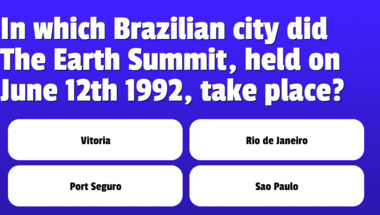The image features a large, horizontally oriented blue rectangle with a quiz prompt in white text. The question reads: "In which Brazilian city did the Earth Summit, held on June 12, 1992, take place?" Beneath the query are four rectangular white buttons arranged in two rows of two, each inscribed with black text featuring potential answers: "Victoria," "Rio de Janeiro," "Porto Seguro," and "São Paulo." The text on the buttons is left-justified, creating a tight alignment emerging almost cut-off on the left side, while a significant negative space on the right showcases more of the vivid blue background. The layout lacks any URLs, branding, or identifiers that might reveal its origin, possibly suggesting its use in trivia related to travel or environmental websites, or as part of an interactive advertisement.